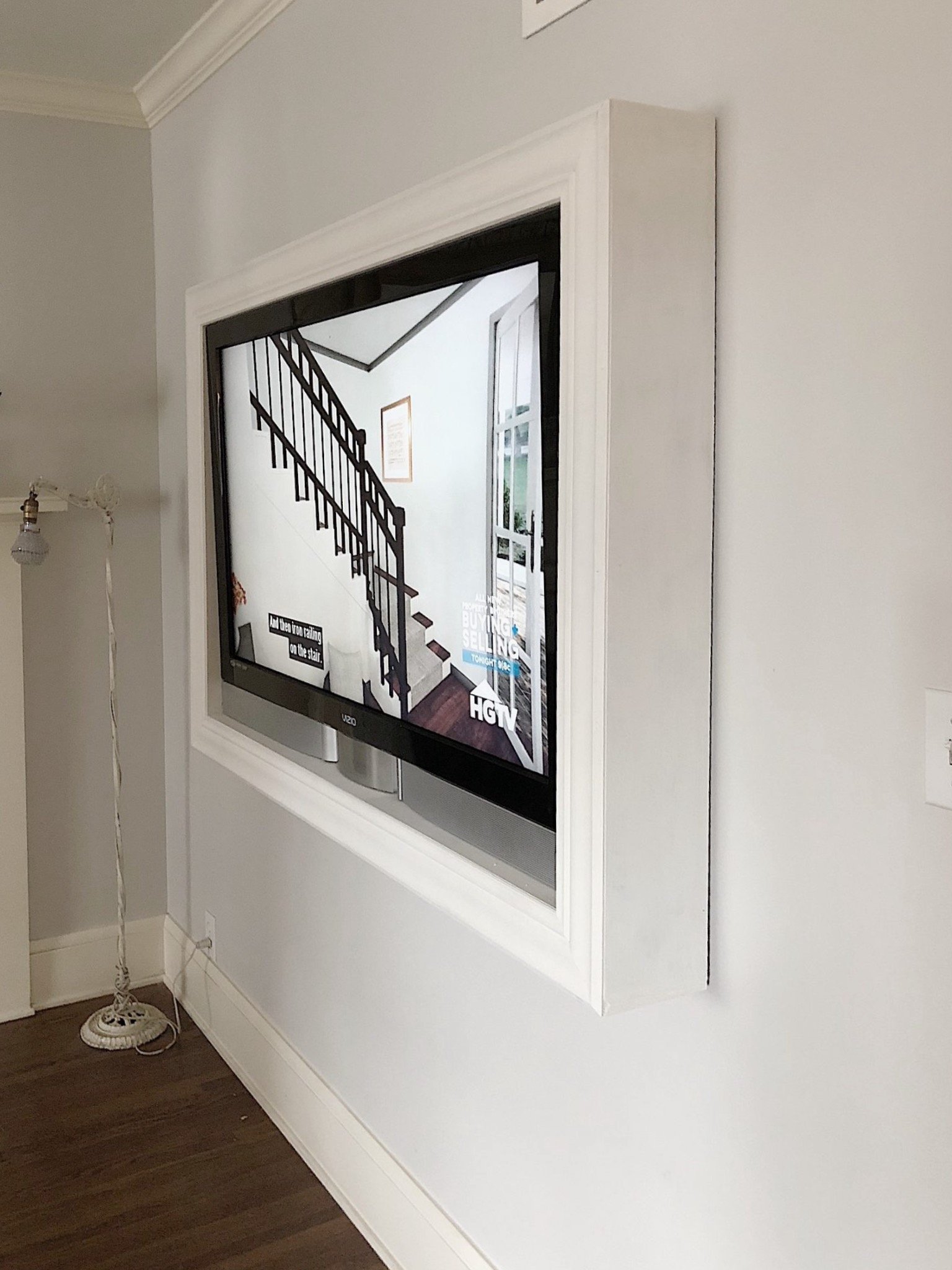The image depicts a cozy indoor living room scene with white walls and rich, dark brown hardwood floors. Centered prominently on the right side, a Vizio TV is mounted on the wall within a protective white frame, giving it an elegant, boxed-in appearance. The TV screen, surrounded by a black border, is tuned into HGTV, displaying an image of a staircase with a wooden guardrail and a grid-patterned full-length window. Superimposed text on the TV screen reads "buying and selling tonight" and "HDTV" in white. Below, partially obscured closed captions appear as black rectangular bars with white text. To the left and slightly towards the center of the image stands a sleek, off-white lamp with a white base and pole. The lamp, which curves and directs light downward, adds to the room's comfortable ambiance. The room's design is completed with white ceiling and light gray or off-white walls, adding to the fresh, clean atmosphere.